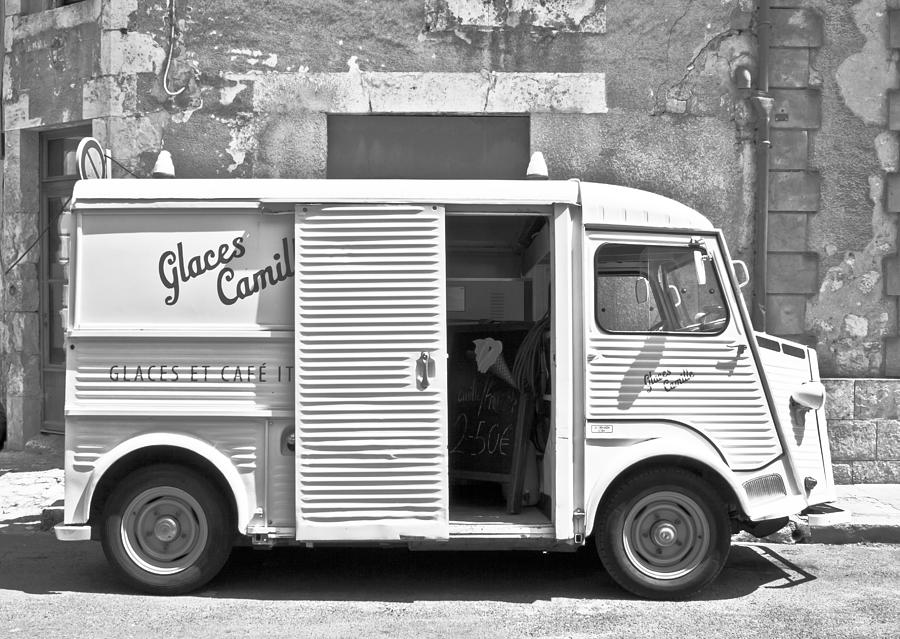This vintage black-and-white photograph captures a nostalgic, old-style ice cream truck with the brand name "Glacis Camille" prominently displayed. The truck, with its horizontal lines and bell mounted near the stop sign, is parked along a shabby, disheveled brick building shaded in various grays, which is showing signs of wear and re-plastering. The side of the truck features faded lettering "Glacis et Café," indicating a possible foreign origin. The vehicle's door is open, revealing a chalkboard with written details inside and a poster advertising ice cream for $2.50. This scene, set beside a rundown structure, evokes a sense of the past with its aged aesthetic and simple charm.